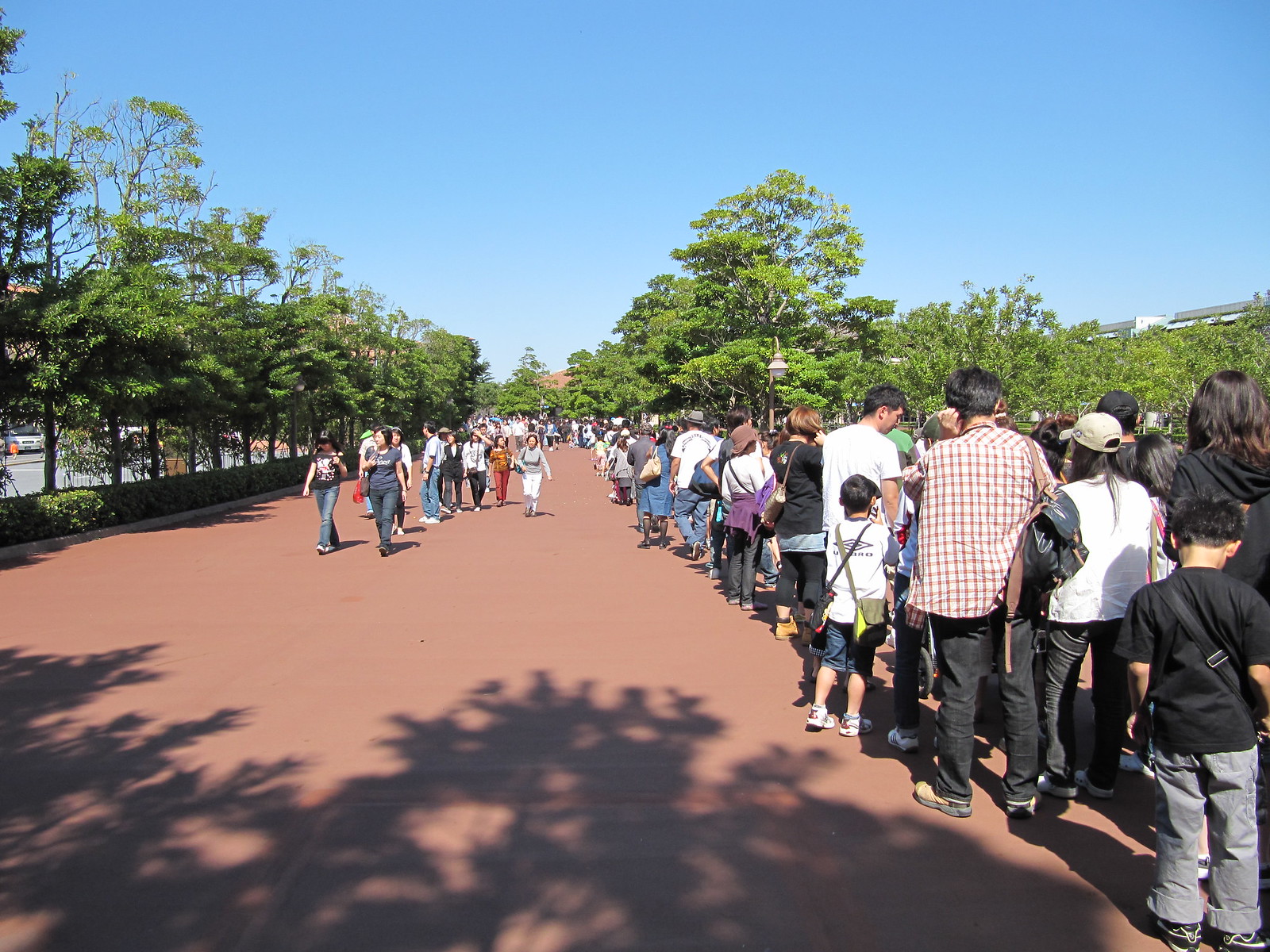The image depicts a wide, brown concrete walkway, potentially in a city park or theme park, bustling with people on a sunny day under a clear blue sky. The scene is dominated by two parallel groups of people: one group consists of hundreds, possibly thousands, of individuals standing in a very long line to the right of the walkway, including men, women, and children of all ages, many wearing backpacks and varying in attire from jeans to shorts, some with hats. The other group includes people walking towards the viewer on the left side of the walkway. The area is flanked by trees and shrubs on both sides, with a parking lot visible beyond the trees to the left and some buildings to the right. The overall composition suggests a busy outdoor event or popular attraction that has gathered a large crowd, resulting in a long line of people waiting for an unknown destination.